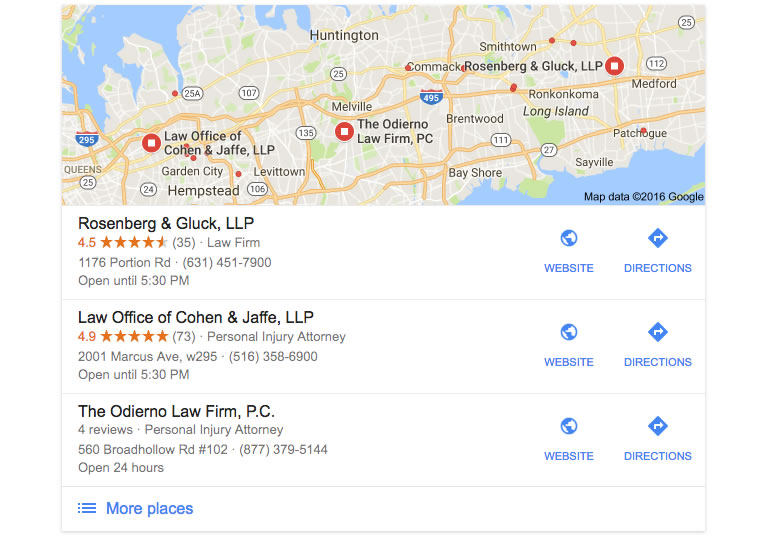The image depicts a detailed map indicating the locations of three law firms in the Huntington area. The map prominently features several towns, including Melville, Garden City, Levittown, Sayville, Bay Shore, and Medford. Below the map, there are search results displaying information about three businesses:

1. **Rosenberg and Kluck LLP**: A law firm with a rating of 4.5 stars based on 35 reviews. The firm operates until 5:30 PM.
2. **Law Office of Cohen and Jaffe LLP**: A personal injury attorney with an impressive rating of 4.9 stars garnered from 73 reviews. This office also remains open until 5:30 PM.
3. **Theodoro Law Firm**: Another personal injury attorney's office. Detailed review and rating information are not specified in the voice caption.

Each firm's exact location is marked on the map at the top of the image. The map primarily focuses on the Huntington area, highlighting other nearby towns and regions for better context.